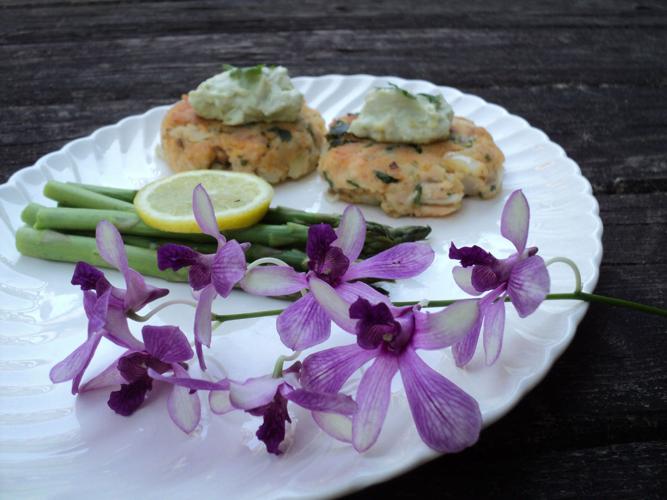In this photograph, a large white plate is prominently displayed on a dark black wooden table. The centerpiece of the plate is a vibrant green bunch of asparagus spears topped with a fresh slice of lemon. Towards the back of the asparagus sit two fried, burger-like crab cakes, each generously topped with a light green sauce, possibly a guacamole or green goddess dressing. In the foreground of the plate lies a delicate branch adorned with purple and white flowers, potentially lilacs or wild onions, their green stem extending gracefully across the dish. This detailed and colorful presentation underscores the appetizing and visually appealing arrangement.